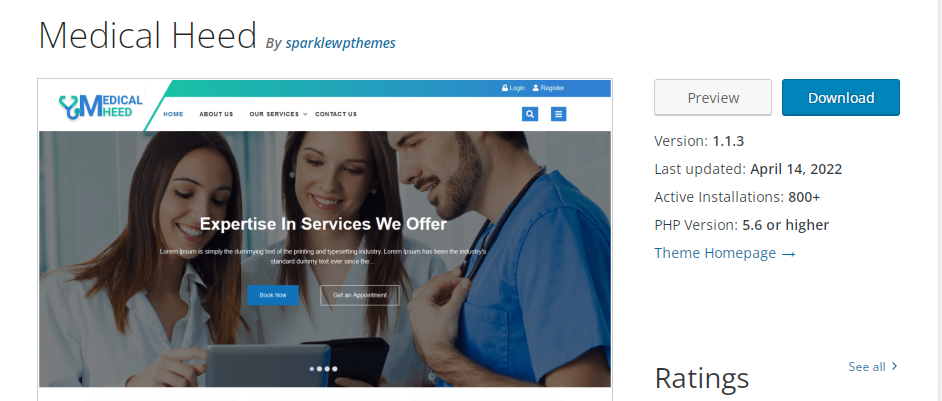The image showcases the header of a website template named "Medical Heed" by Sparkle WP Themes. The "Medical Heed" text is prominently displayed in large, bold black font, while the word "by" is styled in smaller italicized grey text. "Sparkle WP Themes" is written beneath it in blue italics.

Directly below this header is a promotional image likely advertising the website layout. It features a background image of doctors, partially obscured by an overlay module. The module headline reads "Expertise and Services We Offer." Below this, in smaller, light grey text that is somewhat hard to read, it says, "Lyric Morum Ibsen is simply the deforming heart." The call-to-action button on this overlay reads, "Book Morum," in blue text.

To the right side of the overlay, there is additional text detailing the template's specifications and version information, though parts of it are cut off. It includes statements like "Version 1.1.3," "Last updated April 14, 2022," "Active installations 800+," and "PHP version 5.6 or higher." Beneath these details, two blue hyperlinks read "Theme Homepage" and "See All."